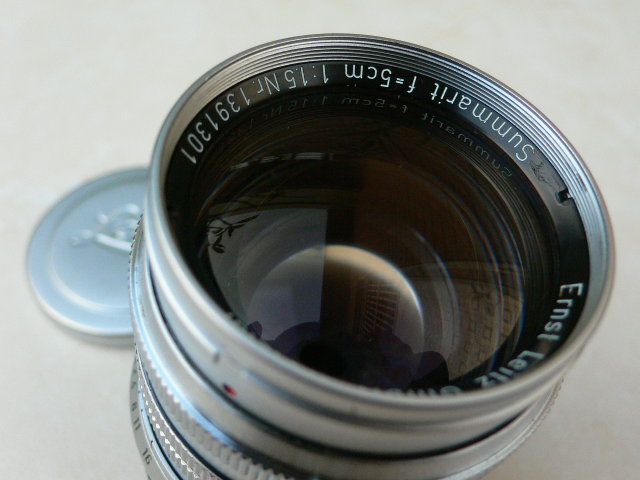This image is a close-up of a cylindrical camera lens standing upright against an off-white background. The lens, which has a reflective glass center, features a metallic outer structure with a silver rim and a black border near the inner glass. On the lens, the text "Ernst Leitz Summarit F=5 CM 1:1.5 NR. 1391301" is visible, detailing its specifications and product number. Behind the lens, a silver lens cap is positioned, and it appears semi-transparent. A red dot is located on the bottom left of the lens. The reflective surface of the lens captures what looks to be square and rectangular shapes, adding to the intricate details of the shot.